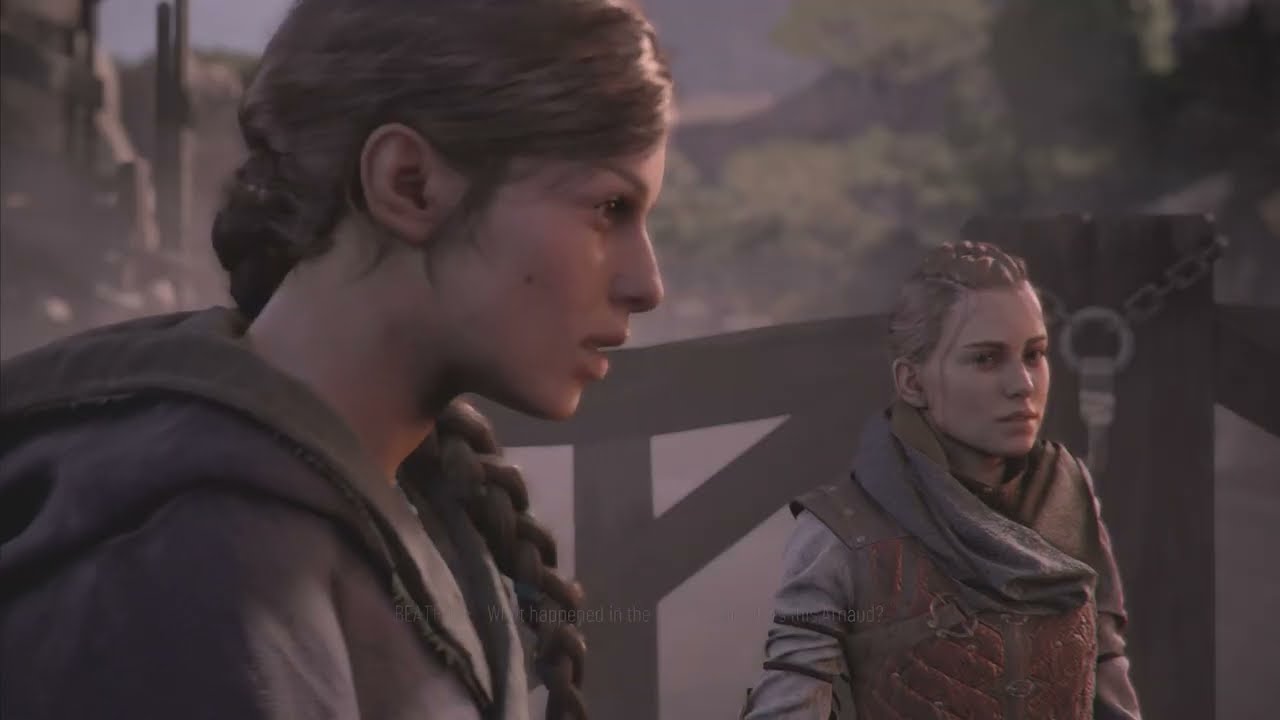The image depicts a highly realistic scene, likely extracted from a video game with detailed 3D graphics. Two women, dressed in medieval-style attire, are standing on what appears to be a wooden bridge or platform with a railing. The scene has a neutral beige and gray tone, complemented by the natural elements such as trees, hills, and mountains in the background.

In the foreground on the left, a young woman with long, light brown or auburn braided hair is shown in profile, looking straight ahead with a neutral expression. She wears a grayish-brown cloak or smock. To the right, another woman stands, slightly further back, gazing into the distance towards the camera. She has light brown or blonde braided hair and is dressed in a medieval vest, possibly accompanied by a scarf, in earthy tones of green and brown. The overall setting evokes a historical or fantasy ambiance, reminiscent of the "Lord of the Rings" era.